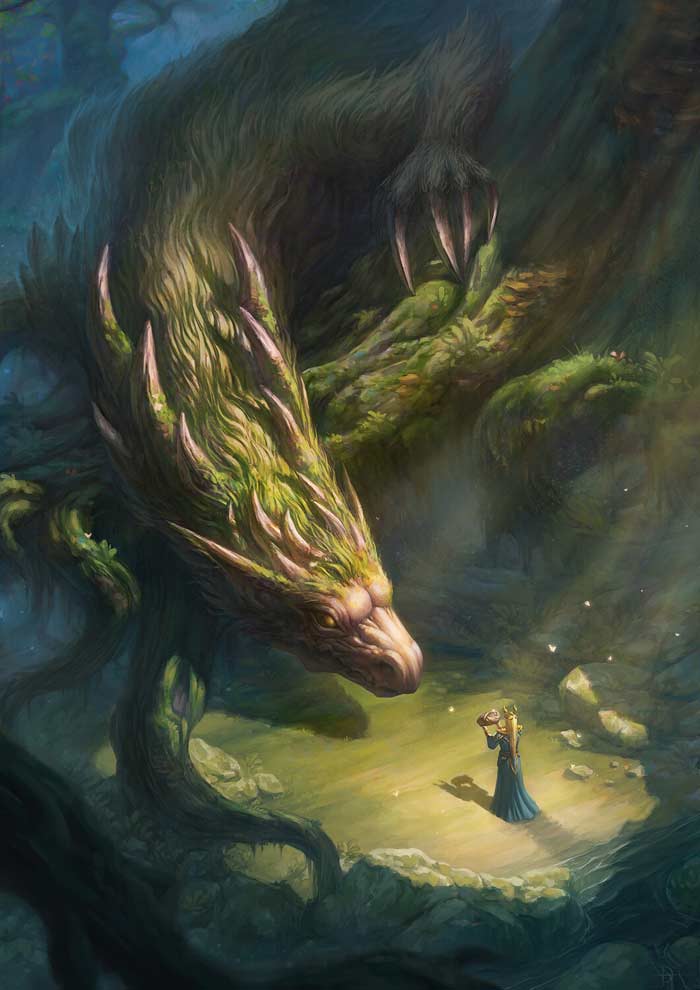The artwork showcases a dramatic scene set within a mythological landscape. On the left side of the painting, a towering dragon dominates the composition with its imposing presence. This creature, vividly rendered in brown tones with a green body, boasts a head adorned with numerous horns and a robust leg that ends in a palm with four sharp, elongated claws. The dragon appears to be partly emerged from the shadows of a cave, adding a sense of mystery and danger to the scene. 

In stark contrast, a woman dressed in a flowing blue gown stands bravely before the dragon. Her blonde hair catches the light that pierces through the dense forest canopy, suggesting it is daytime. She holds out a parcel, seemingly as an offering or a gift to the dragon, infusing the composition with a sense of narrative tension. Tall trees with sprawling roots frame this fantastical encounter, enveloping both figures in an aura of enchantment and suspense. The overall atmosphere of the painting blends mythical elements with rich, detailed imagery, capturing a moment ripe with potential conflict or alliance.